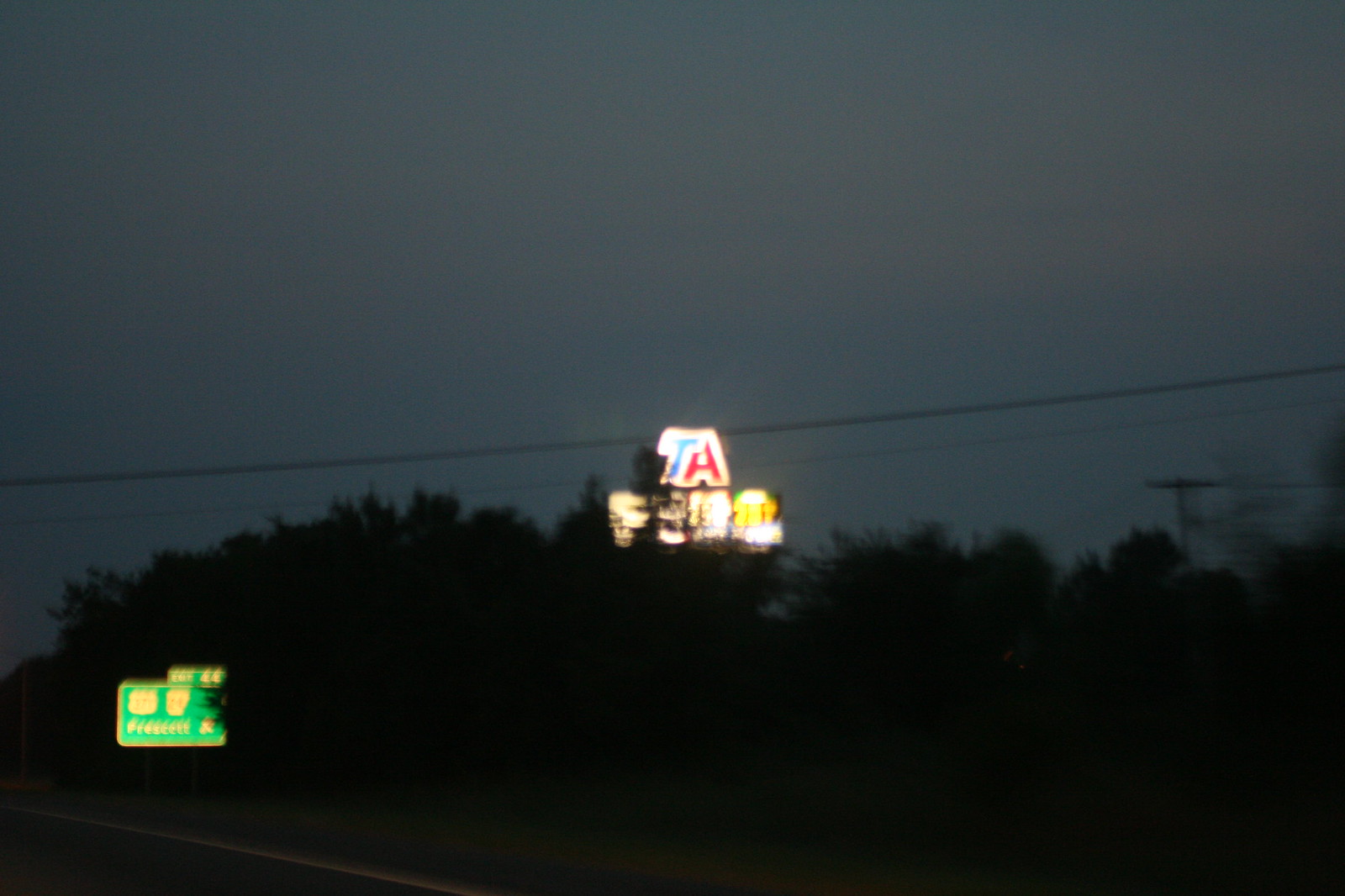The photograph captures a scene from a moving car on a highway, depicted during the transitional light of either dusk or dawn. The sky retains a subtle illumination despite being predominantly dark, creating a serene backdrop. In the distance, a silhouette of trees is intermittently interrupted by power lines. A prominent feature in the image is a large sign for a truck stop, with a distinctive blue "T" and red "A," identifying it as a Travel Centers of America location. Below the sign, the gas prices are visible but blurred, rendering the specific numbers unreadable. In the lower left corner of the image, a green highway sign indicates "Exit 44," accompanied by both a state route and a U.S. route logo, along with an arrow pointing towards an unreadable city name and route numbers. The photograph is a representation of a typical highway scene, marked by familiar navigational and commercial signs seen by many travelers.